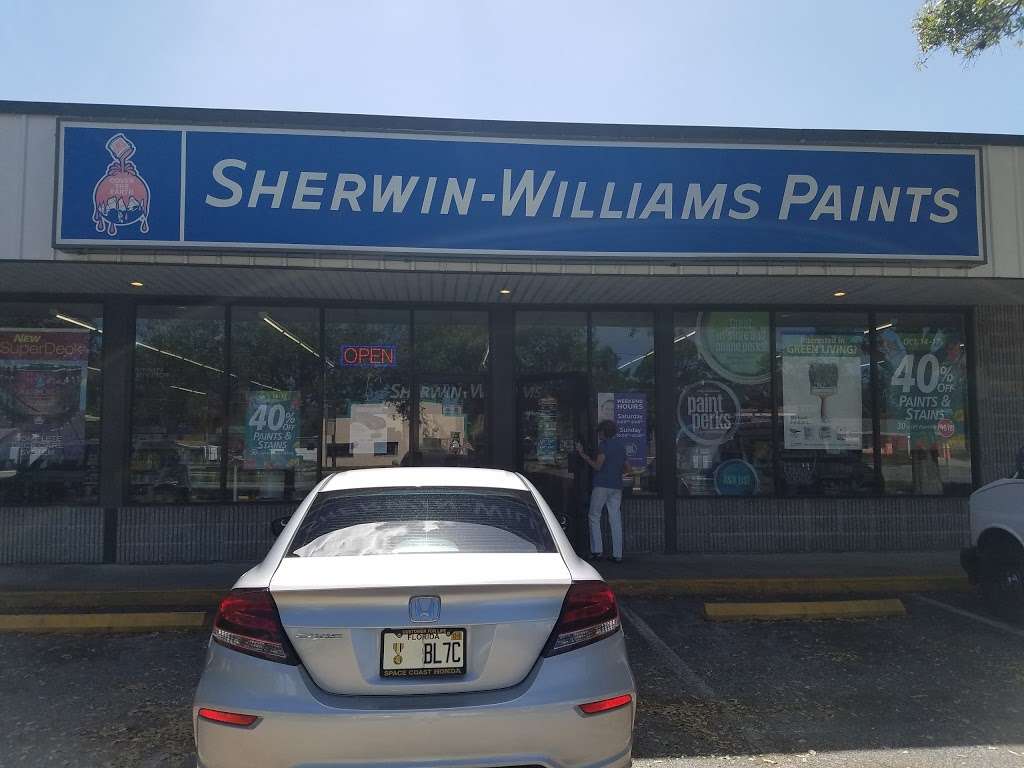A vivid photograph captures the front exterior of a Sherwin-Williams paint store on a clear day with a bright blue sky. A silver Honda, bearing a Florida license plate reading 'BL-7C,' is parked directly in front of the store. A person, dressed in a short-sleeved blue shirt and white pants, is entering the store through the front door. To the far right, the edge of a white vehicle, likely a van, is just visible. The store’s "Open" sign is illuminated in the window. A large poster featuring a paintbrush is displayed on the far right side of the store next to a sign announcing a 40% discount on paints and stains. There are four clearly defined parking spots visible in the scene.